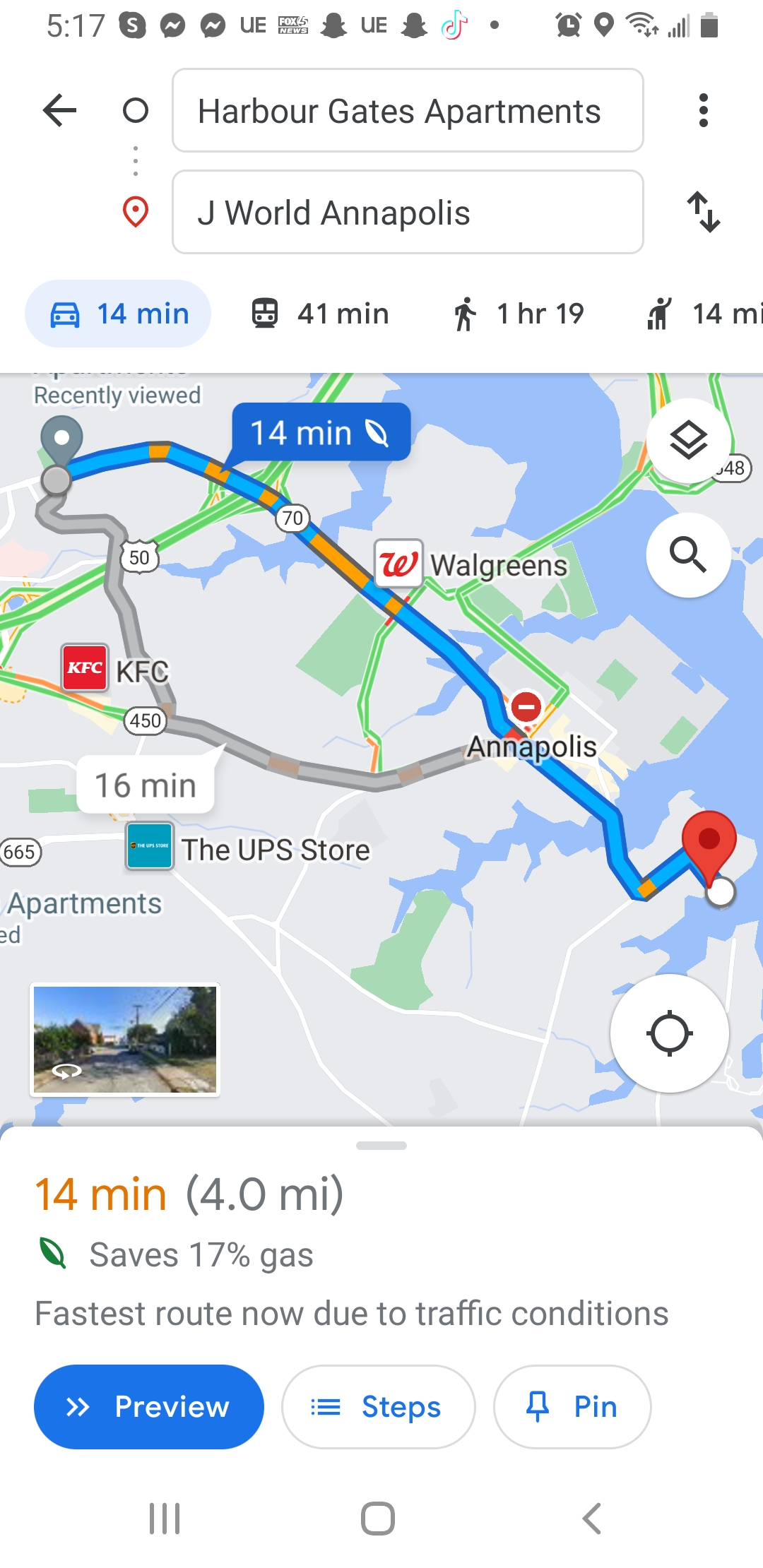This image is a detailed navigational map, likely from Google Maps or a similar mobile application, showing the route from Harbor Gates Apartments to J World Annapolis. The top of the map indicates a 14-minute drive covering a distance of 4.0 miles, saving 17% on gas and being the fastest route due to current traffic conditions. The path is color-coded, with yellow indicating denser traffic and blue indicating lighter traffic. Key landmarks along the route include a Walgreens, KFC, and a UPS store. Alternative travel options are also highlighted: 41 minutes by train, 14 minutes by taxi, and 1 hour and 19 minutes on foot. At the bottom of the map, there is a blue "Preview" button, followed by options labeled "Steps" and a pin icon. The lower left-hand corner features a small inset photograph, which is difficult to distinguish but could potentially be either the starting point or the destination.